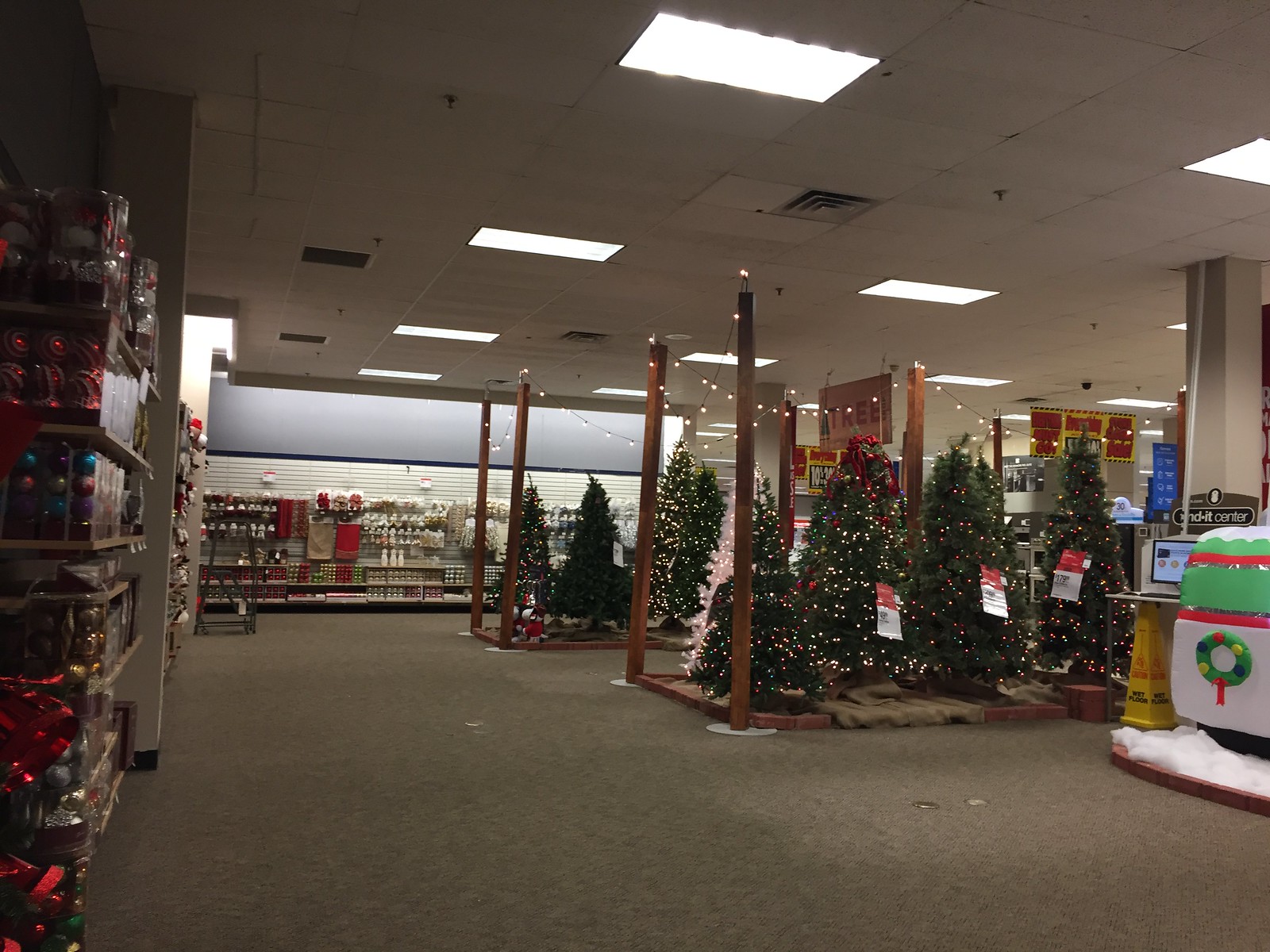The image captures the Christmas section of what appears to be a department or specialty store, characterized by its gray carpet flooring and white tiled ceiling with rectangular fluorescent lights and integrated fire sprinklers. The focal point is a neatly arranged display of around ten Christmas trees, mostly green with one strikingly white, all adorned with lights. Three trees on the right side feature red and white price tags, though the prices are not legible. The left and back walls showcase neatly organized ornaments and Christmas decorations, displayed on lap board siding and stacked on five wooden shelves. Snow-like decor and wooden posts with party lights add festive touches, enhancing the holiday ambiance. The perspective suggests the photo was taken from a standing position near the left wall, capturing a detailed, immersive view of the store's festive offerings.